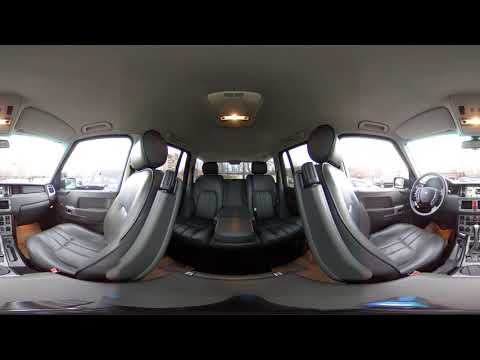The image is a highly distorted panorama, capturing the interior of a car, likely taken with a 360-degree camera. The photograph merges multiple angles, creating a warped perspective where the passenger seat appears on the far left, oriented towards the left, and the driver's seat is on the far right, facing right. Centrally, the two back seats are visible, separated by a folded-down console that gives the illusion of a third seat being absent. The interior upholstery is a uniform gray, resembling faux leather, and appears clean with no visible clutter. The steering wheel is in front of the driver's seat, accompanied by the front dash, shifter, and an overhead console. The vehicle's roof is visible with the central interior light turned on. Despite the distortion, it’s evident that the image was taken during the daytime, as bright natural light floods in through the windows, though the outside scenery remains indistinct.